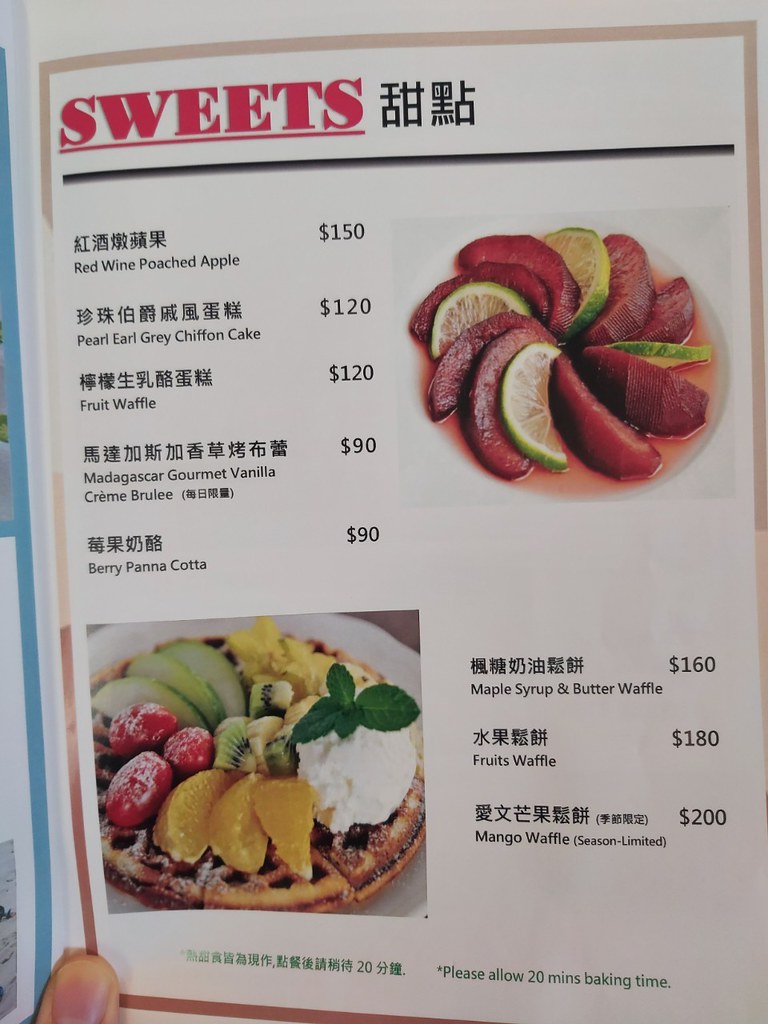In the image, someone is holding a paper menu, partially written in what appears to be Mandarin or Chinese, alongside English text. The person's thumb is visible in the binding part of the menu. At the very top of this section, the word "SWEETS" is prominently displayed in all red capital letters, juxtaposed with the foreign language equivalent next to it.

The menu features a variety of desserts, with some astounding prices which suggest it might be a catering menu. Notably, there's "Red Wine Poached Apple" priced at $150 and "Pearl Earl Grey Chiffon Cake" for $120. Both items are listed with their names in the foreign language directly underneath.

On the bottom left of the image, there is a picture of a waffle garnished with various fruits. The waffle is accompanied by a side of maple syrup and butter, listed on the menu as costing $160. This particular waffle features cottage cheese and segments of mandarin oranges or peaches, along with raspberries and other unidentified fruits. It likely corresponds to the "Fruit Waffle" item priced at $180, with a note indicating a 20-minute baking time.

Additionally, there are images of other desserts on the menu, such as a Madagascar Gourmet Vanilla Crème Brûlée and a Berry Panna Cotta. One dessert features an arrangement of lime and other fruits, with a reddish juice at the bottom, possibly representing the "Red Wine Poached Apple." The whole assortment adds a vibrant and visually appealing touch to the glamorous yet pricey menu.